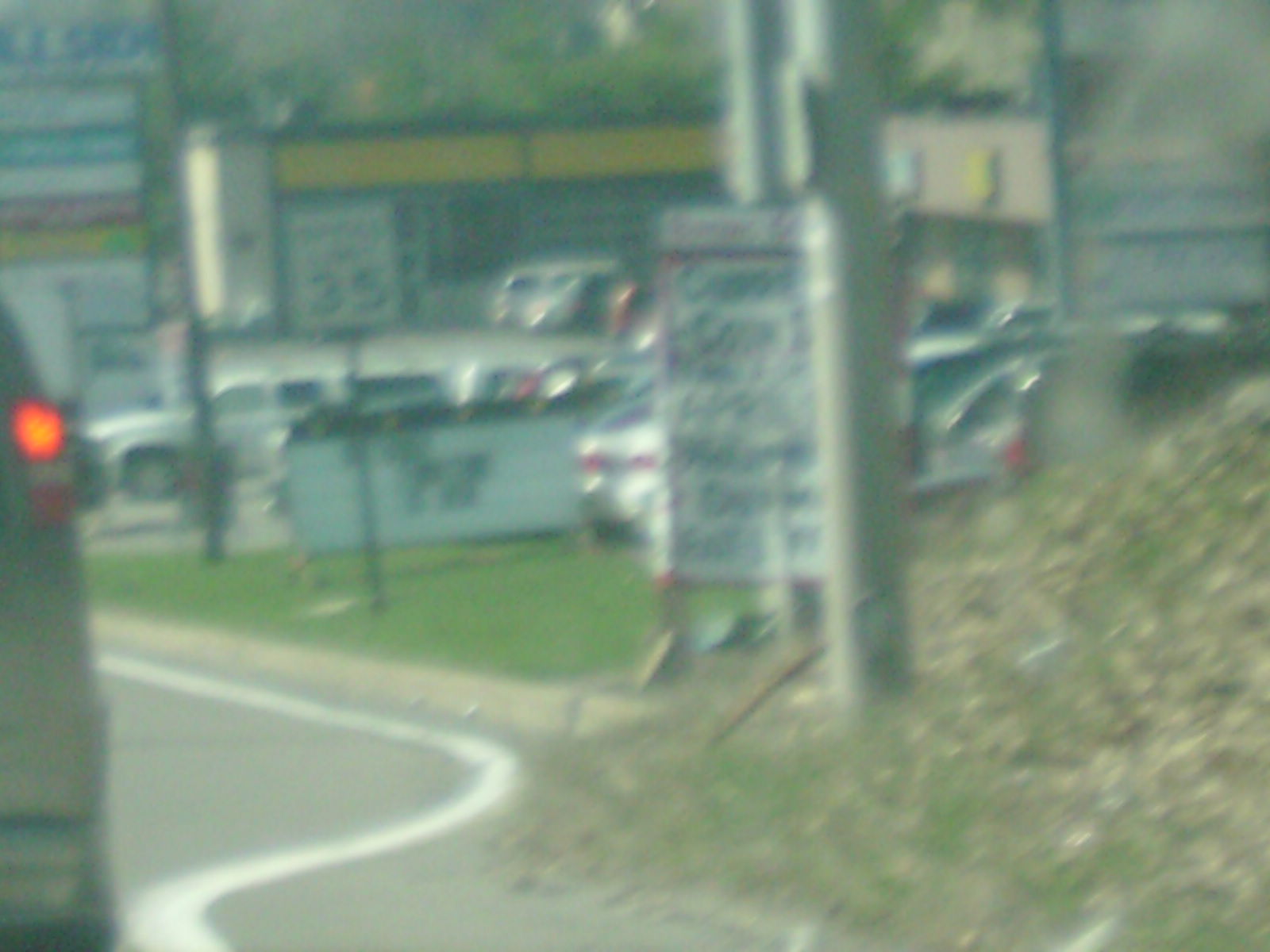In this blurry, low-resolution photograph taken in daylight from a car in traffic on a winding road, several detailed elements are visible despite the lack of clarity. To the left, a person's leg and tan shoe are visible next to an illegible handwritten sign advertising a business. A marquee sign with light bulbs and black text is prominently positioned behind this individual, set amid a small shopping plaza or service area with potential shops and fast food places. Center-left is a speed limit sign indicating 35 mph. The roadway curves to the right, leading to an intersection, with cars populating the parking lot around the plaza. At the top of the photo, a yellow banner or walking bridge is visible, while a grassy hill rises to the right. Additionally, the tail light of another car is visible at the bottom left corner of the image.